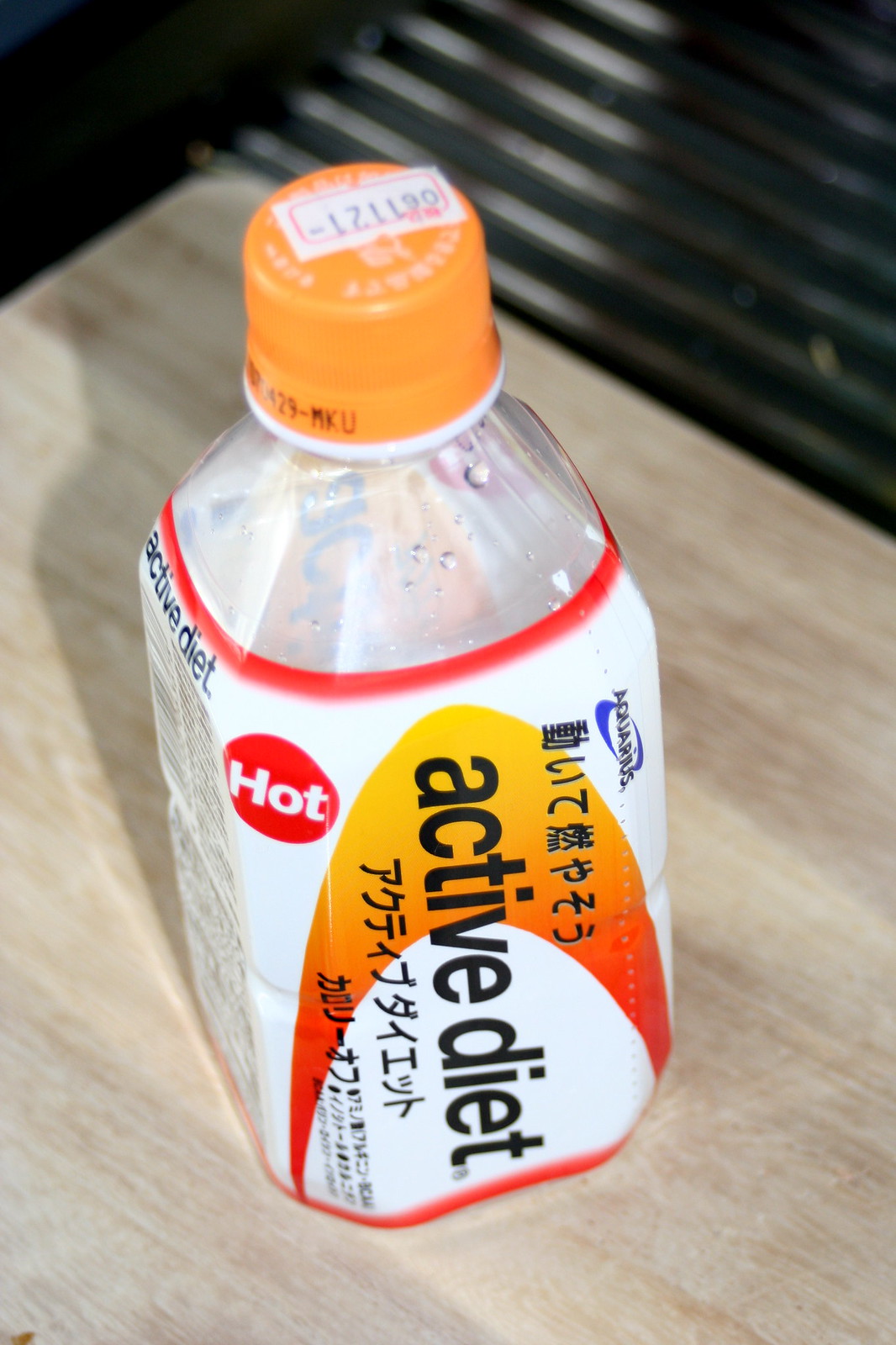This indoor photograph centers on a small plastic bottle placed prominently on a light brown wooden surface. Adjacent to the wood is a darker metallic surface featuring hues of dark blue and silver. The bottle, which is the main focus, has a vividly designed label dominated by red, white, and yellow colors. The label prominently displays the text "Active Diet" and features a distinct red circle with white lettering that reads "HOT." Additionally, the label is adorned with numerous Japanese characters, adding an international flair. The bottle is capped with an orange lid, topped with a white sticker. Although the bottle appears to have condensation on the interior, it might actually be empty. The composition of the image highlights the contrast between the warm wooden surface and the cool metallic tones, framing the colorful and eye-catching bottle perfectly.